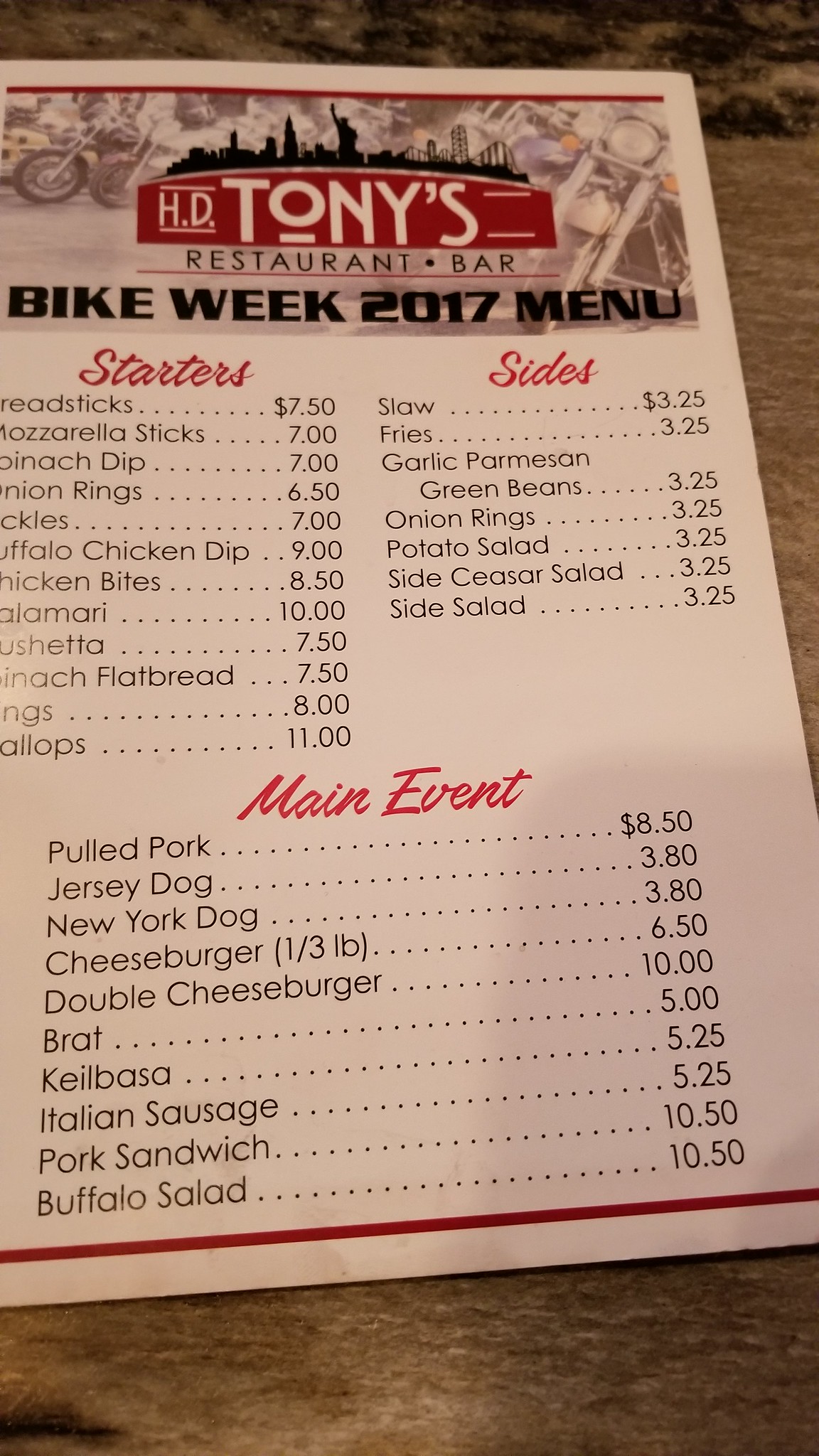This photo captures a menu from HD Tony's Restaurant and Bar during Bike Week 2017. The menu is organized into three main sections: Starters, Sides, and Main Event.

In the **Starters** section, although some items are partially cropped, the visible items include:
- Breadsticks
- Mozzarella Sticks
- Spinach Dip (partially cropped)
- Onion Rings (partially cropped)
- Buffalo Chicken Dip (partially cropped)
- Calamari (partially cropped)
- Bruschetta (partially cropped)
- Spinach (partially cropped)
- An item presumed to be Scallops (partially cropped)

Prices for the starters range from $6.50 to $11.00, indicated with dotted lines separating the items and their respective prices.

The **Main Event** section features a variety of hearty dishes, each neatly paired with its price:
- Pulled Pork
- Jersey Dog
- New York Dog
- Cheeseburger (one-third pound)
- Double Cheeseburger
- Brat
- Kielbasa
- Italian Sausage
- Pork Sandwich
- Buffalo Salad

Finally, the **Sides** section offers additional options to complement the main meals:
- Slaw
- Fries
- Garlic Parmesan
- Green Beans
- Onion Rings
- Potato Salad
- Side Caesar Salad
- Side Salad

Each section is clearly laid out with a logical flow, allowing for an easy and enjoyable browsing experience for patrons.